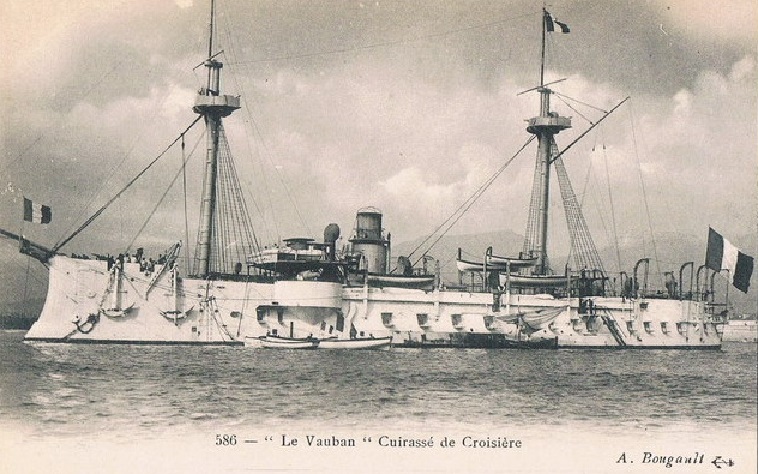This black-and-white photograph depicts an old steamship named "Le Vauban," stretching horizontally across the entire frame. The ship, with a flat hull painted white, features two tall masts equipped with bird's nests and supporting cables, as well as a prominent chimney in the middle, suggesting it is a steam-powered vessel. At the fore and aft of the ship, there are large flags with three vertical stripes, consistent with the French flag's design, and the text on the image is also in French.

The vessel is adorned with several visible features including windows cut out towards the aft, cannon or guns protruding through portholes along its sides, and superstructures located just behind the front mast and further towards the back. Notably, at the top of each mast is a platform with slender poles extending upwards, one of which carries a flag.

In the foreground, the photo captures the ocean's waves against the ship's hull, while the background reveals cloudy skies and faint, gray mountains. The aging of the photograph lends a yellowed tint to the otherwise monochromatic scheme.

At the bottom of the image, black print reads "586 - Le Vauban Cuirassé des Croisières," indicating the ship's name and classification, alongside the photographer's name, "A. Bugault," inscribed in the lower right-hand corner.